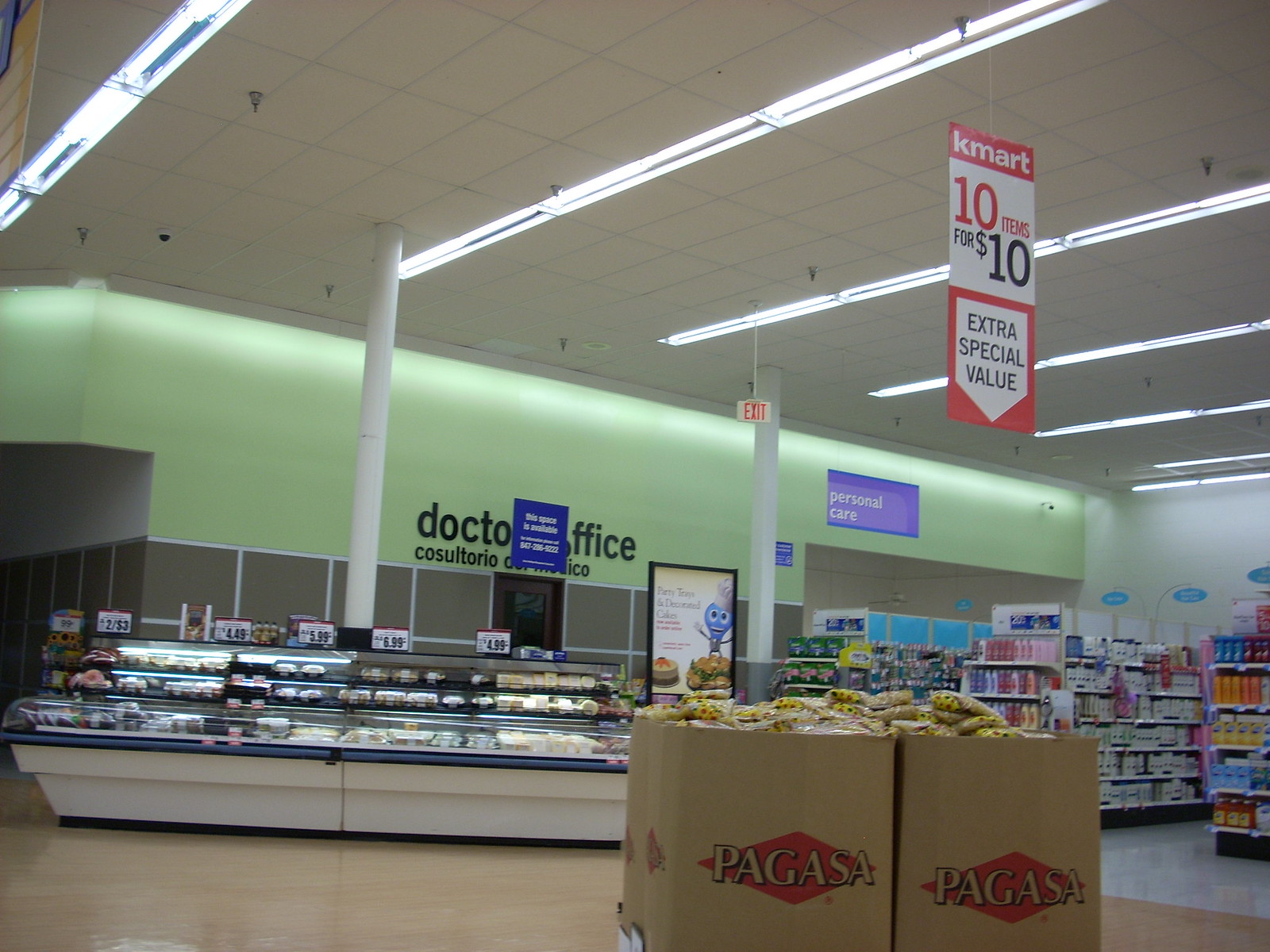The image captures the interior of a Kmart retail store. Prominently hanging from the ceiling is a red, white, and black sign displaying "Kmart" in white lowercase letters against a red background. Below, the sign advertises "10 items for $10," with an arrow pointing downwards that reads "extra special value." 

In the mid-aisle, there is a pallet-like display featuring two cardboard boxes labeled "Pagasa" with a red diamond logo on the outside, containing what appear to be sacks of yellow and beige potatoes. 

Towards the background, there is a refrigerated section and an area that seems to offer fresh foods, possibly including bakery, deli items, and cheese. Detailed grocery prices, such as $4.99 and $6.99 per pound, are also visible. A blue sign overhead proclaims that the adjacent space, labeled “doctor's office” in both English and Spanish, is available for lease.

On the right-hand side, there is a section dedicated to personal care items, indicated by a sign, and stocked with products such as shampoo and body wash, including VO5 brand shampoo and conditioner.